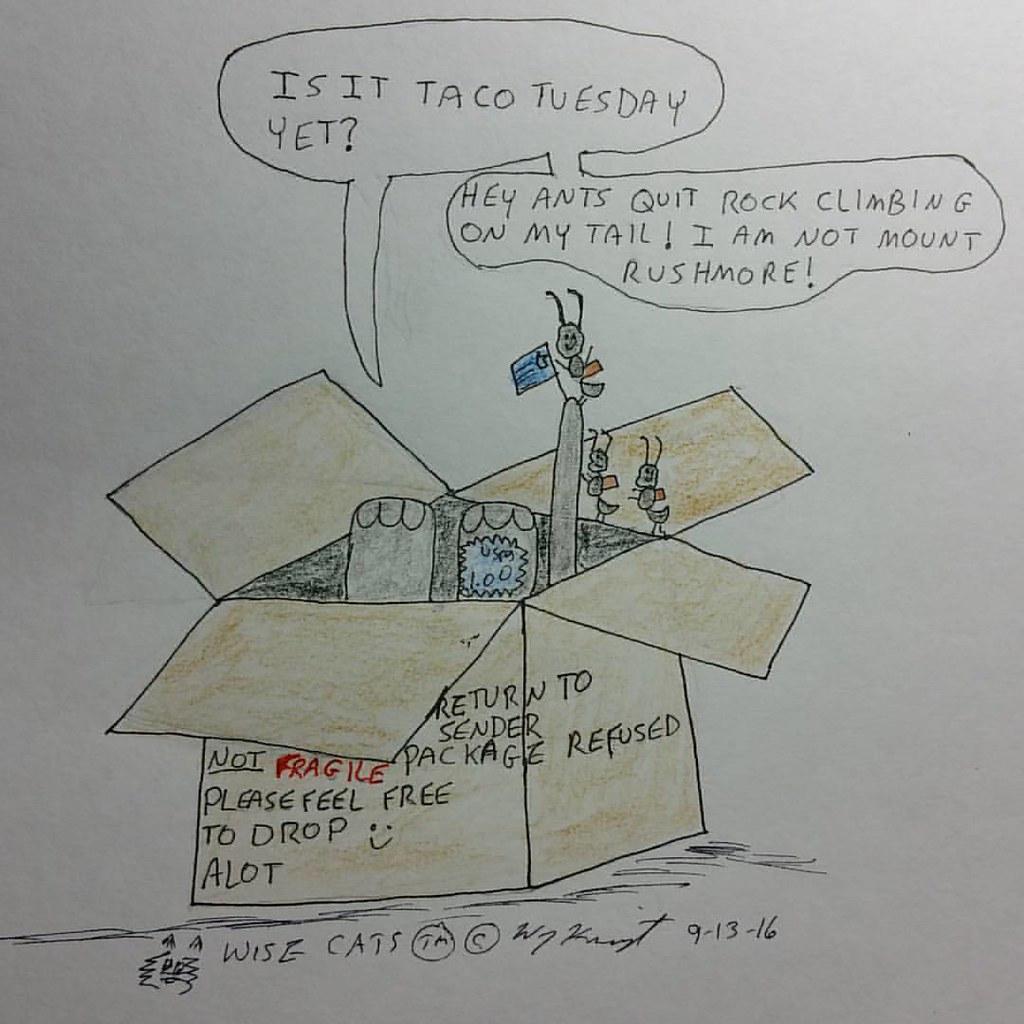This is a photograph or scan of a hand-drawn cartoon, likely created by a child given the primitive style of the drawing and text. The cartoon features a haphazardly drawn cardboard box with cartoonish elephant legs, a tail, and paws sticking out of it. Inside the box are speech bubbles saying, "Is it Taco Tuesday yet?" and "Hey ants, quit rock climbing on my tail. I am not Mount Rushmore." On the tail, three ants are depicted climbing and attempting to plant a flag. The box is labeled with humorous text including "USA $1," "Return to sender," "Package refused," and "Not fragile, please feel free to drop" accompanied by a smiley face. At the very bottom, the drawing is signed "Wise Cats TM," along with a copyright symbol and a signature dated 9-13-16, with an added scribble of a cat next to the text.